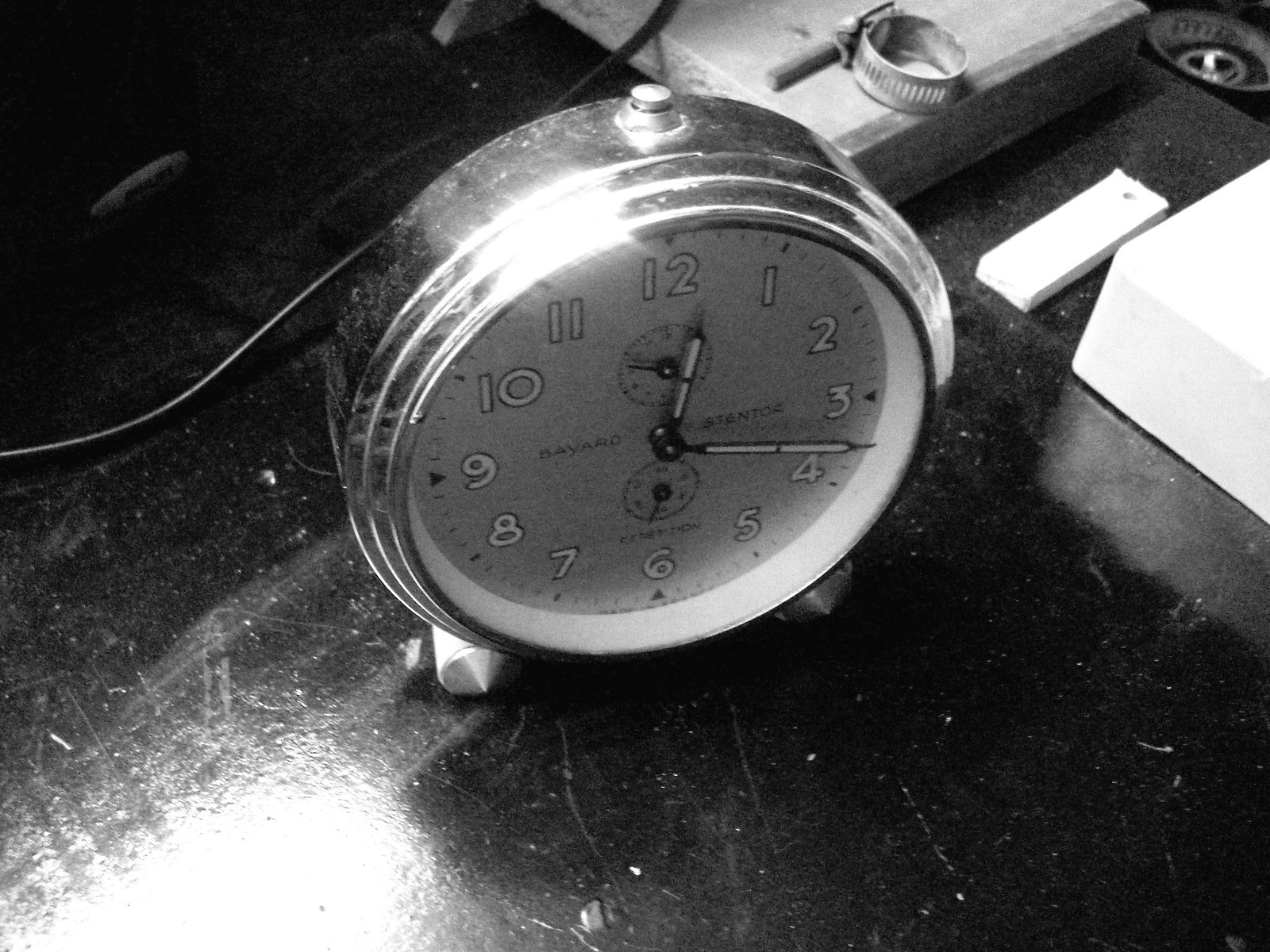This black and white image features a standing clock with a classic design. The clock face, although colorless, displays clearly defined Arabic numerals ranging from 1 to 12, and it has both an hour and a minute hand. The clock is positioned on a dark wooden desk, the exact hue of which is indeterminable due to the monochromatic nature of the image. In the top right corner of the photograph, there appears to be a portion of a tool or mechanism, adding an element of intrigue and suggesting a setting that might be related to craftsmanship or repair.